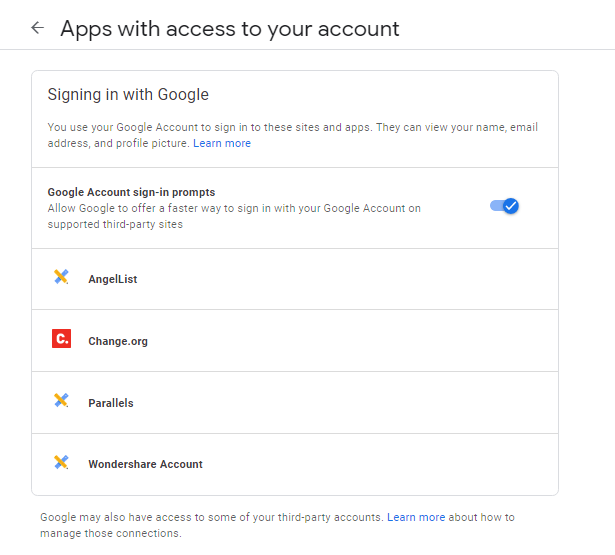The image depicts a Google Account Settings page, specifically focused on the section for "Apps with access to your account." The user interface is characterized by a clean, white background with gray borders and lines that separate different sections and items. 

At the top of the page, there's a heading titled "Apps with access to your account: Sign in with Google." This section explains that users can utilize their Google account to sign in to various sites and apps, allowing these services to view information such as the user's name, email address, and profile picture. Information about account sign-in prompts is also provided here.

Beneath this header, there's a toggle switch that allows users to turn the "Sign in with Google" feature on or off.

The subsequent section lists the apps and websites that currently have access to the account. In this particular instance, the list includes:
1. AngelList
2. Change.org
3. Parallels
4. Wondershare

Each app is listed with a gray dividing line in between, providing clear separation and organization.

At the bottom of the page, there's a note stating, "Google may also have access to some of your third-party accounts. Learn more about how to manage those connections." The text "Learn more" is a clickable hyperlink for users seeking additional information.

This configuration hints that the image could be from the settings of a Google account or possibly from within the settings on a Chromebook, given its familiar layout.